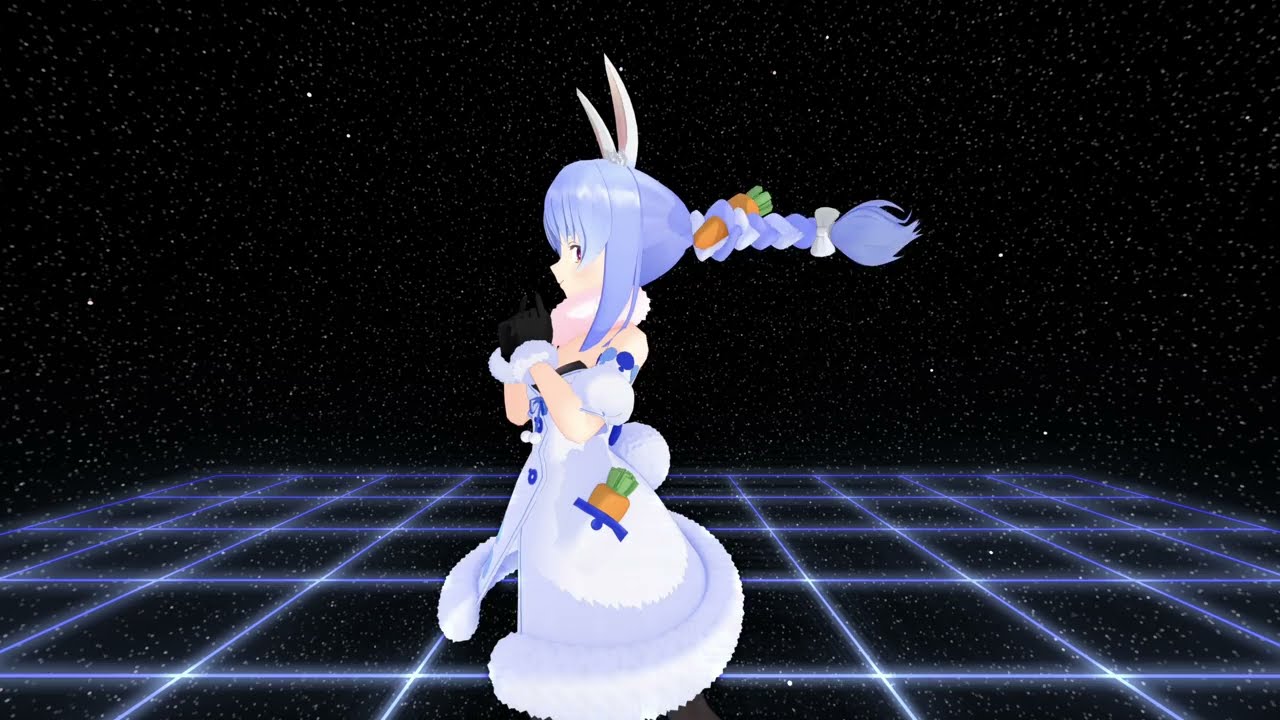This is a screenshot from an anime-style game, featuring a highly detailed caricature set in outer space. The background is pitch black with scattered white specks resembling stars, enhancing the sci-fi and cyber-like atmosphere. The scene's floor is constructed from bright, glowing bluish-whitish laser lines, creating an intricate chessboard-like grid extending both forward and sideways.

At the center of the image stands a young girl, possibly a teenager, with a striking presence. She has light blue hair styled in a primary braid that appears weightless, floating outward behind her head. Integrated into the braid is a curious detail—a carrot, along with a white bow at the end, adding whimsical charm. Loose strands of hair frame her face, which features dark eyes, dark eyebrows, and a pointy nose. Completing her look are a pair of white bunny ears perched atop her head, further reinforcing the bunny girl motif.

She is wearing a flowing light blue gown, adorned with royal blue accents and buttons, which billows gracefully around her. Her hands are delicately folded in front of her chest, suggesting a serene demeanor. Peeking out from her left side pocket is a partially visible carrot, hinting at her playful nature. The overall composition and the character's detailed depiction contribute to a vividly imaginative and engaging scene in the realm of manga and anime illustration.